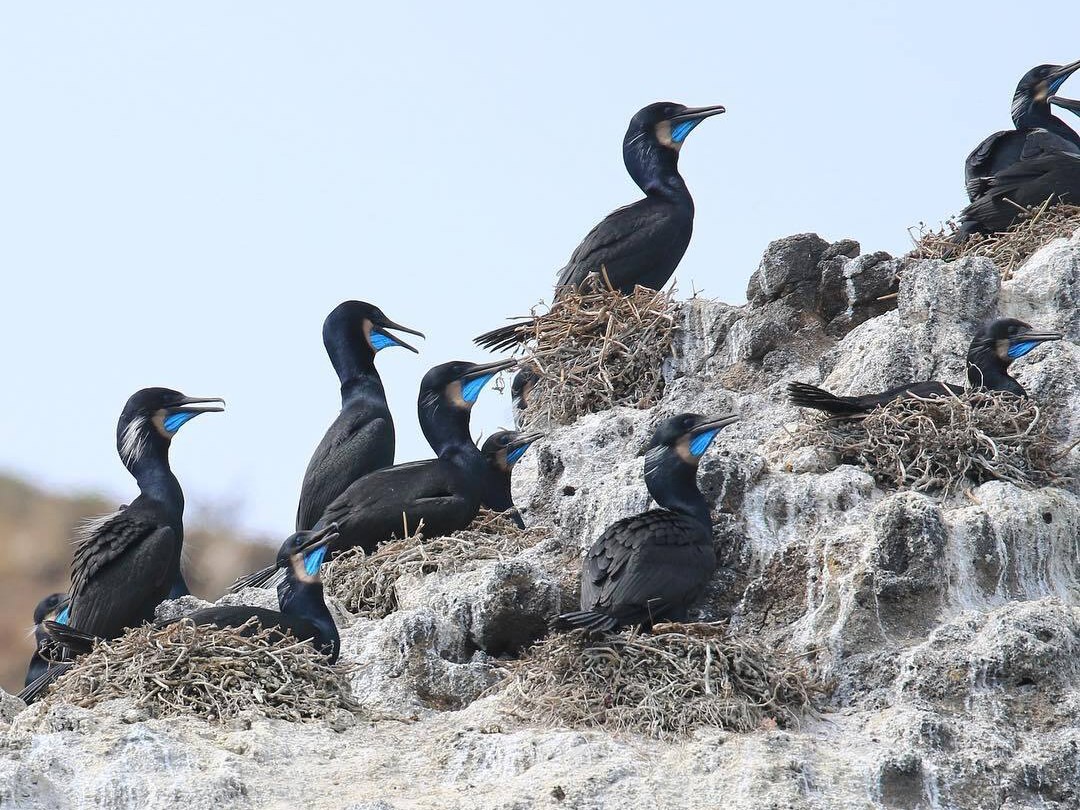In the photograph, a multitude of black seabirds with smooth, dark feathers and vivid light blue throats, accented by touches of white under their chins, are perched on a grayish dirt mound. This dirt mound, resembling a cliff or beach setting, is dotted with several nests made from twigs and sticks, suggesting it is home to these birds. The mound cascades upward from the bottom left corner to the upper right edge of the image and is layered with small levels, making it an intriguing structure. All the birds are uniformly facing to the right, some standing, some sitting, adding a sense of uniformity to the scene. Above them, a bright, light blue sky stretches across the background, reinforcing the natural, outdoor setting. The photograph is slightly wider than it is tall, capturing the serene yet bustling environment of these captivating birds in great detail.